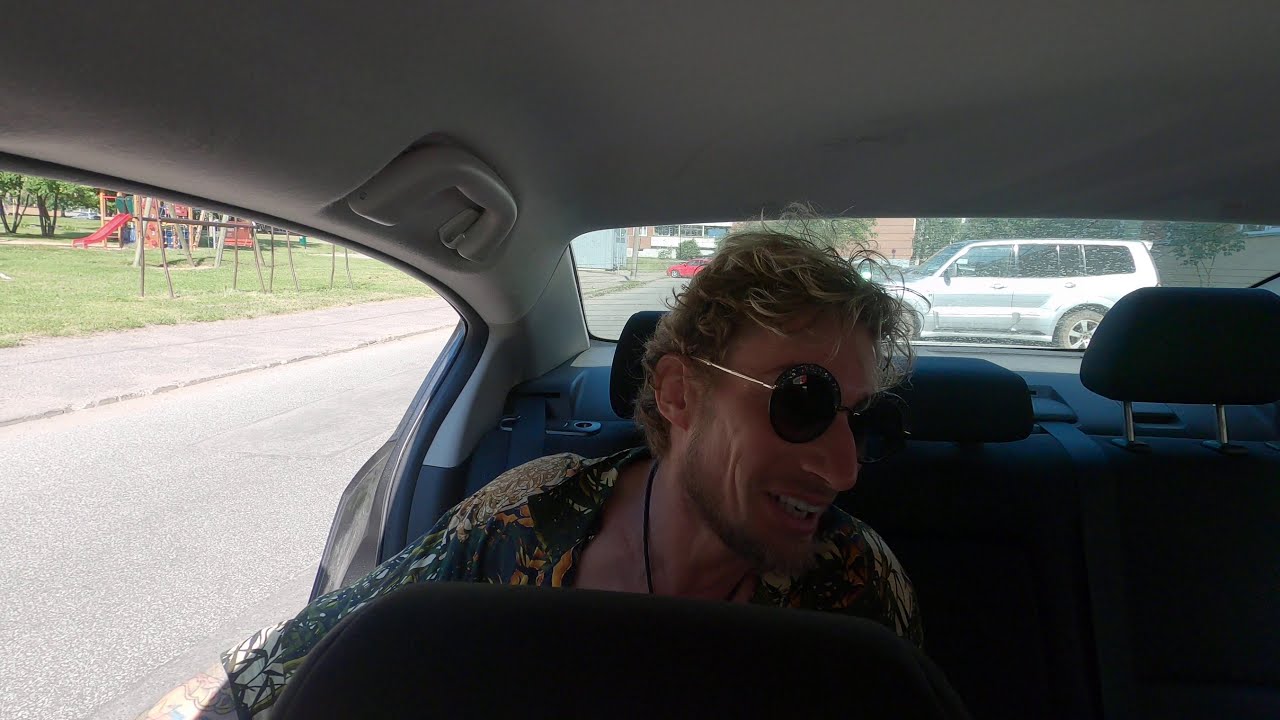In this image, we see the backseat of a passenger car in a bright, daytime setting. The interior roof of the car is gray with dark blue or black fabric seats. Occupying the backseat is a middle-aged man with bleached blonde hair showing dark roots, wearing dark sunglasses with narrow metallic frames. He is dressed in a vibrant, multi-colored Hawaiian floral shirt, predominantly blue, green, and yellow, open at the collar, revealing a necklace. The man, who seems to be smiling, has noticeable stubble and a prominent nose, and he appears to be leaning forward, possibly engaging with someone in the front seat.

Through the car's left side window, an open door reveals a park filled with green grass, slides, and swings. The outdoor setting includes a visible red slide. Behind the car, seen through the rear windshield, various parked vehicles are evident, including a prominent silver SUV and a red car further away. The backdrop also features trees and some brick buildings with visible windows, reinforcing the scene's bright, sunny atmosphere in a residential area.